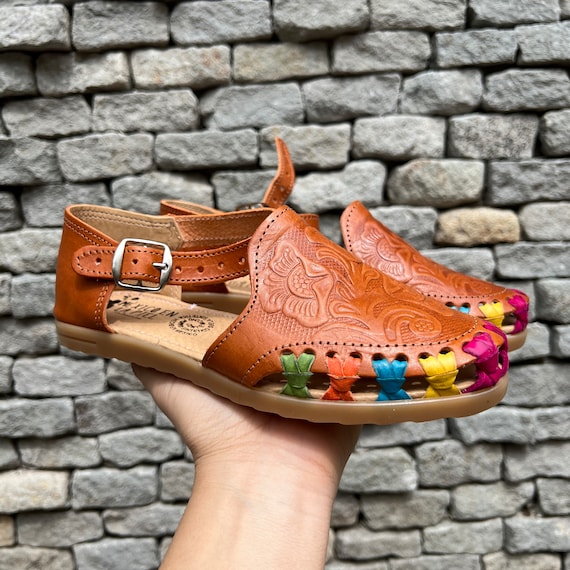This photograph captures a close-up of a person's left hand holding a pair of brown leather sandals up in front of a neatly constructed brick stone wall. The sandals are intricately designed with a floral pattern on the top and feature colorful stitching around the toe area, incorporating green, orange, blue, yellow, and purple ribbons. The sandals also have a buckle on the side and resemble moccasins with a flat sole. The detailed craftsmanship of the shoes, combined with the textured background of the gray brick wall, creates a visually compelling and richly detailed image.